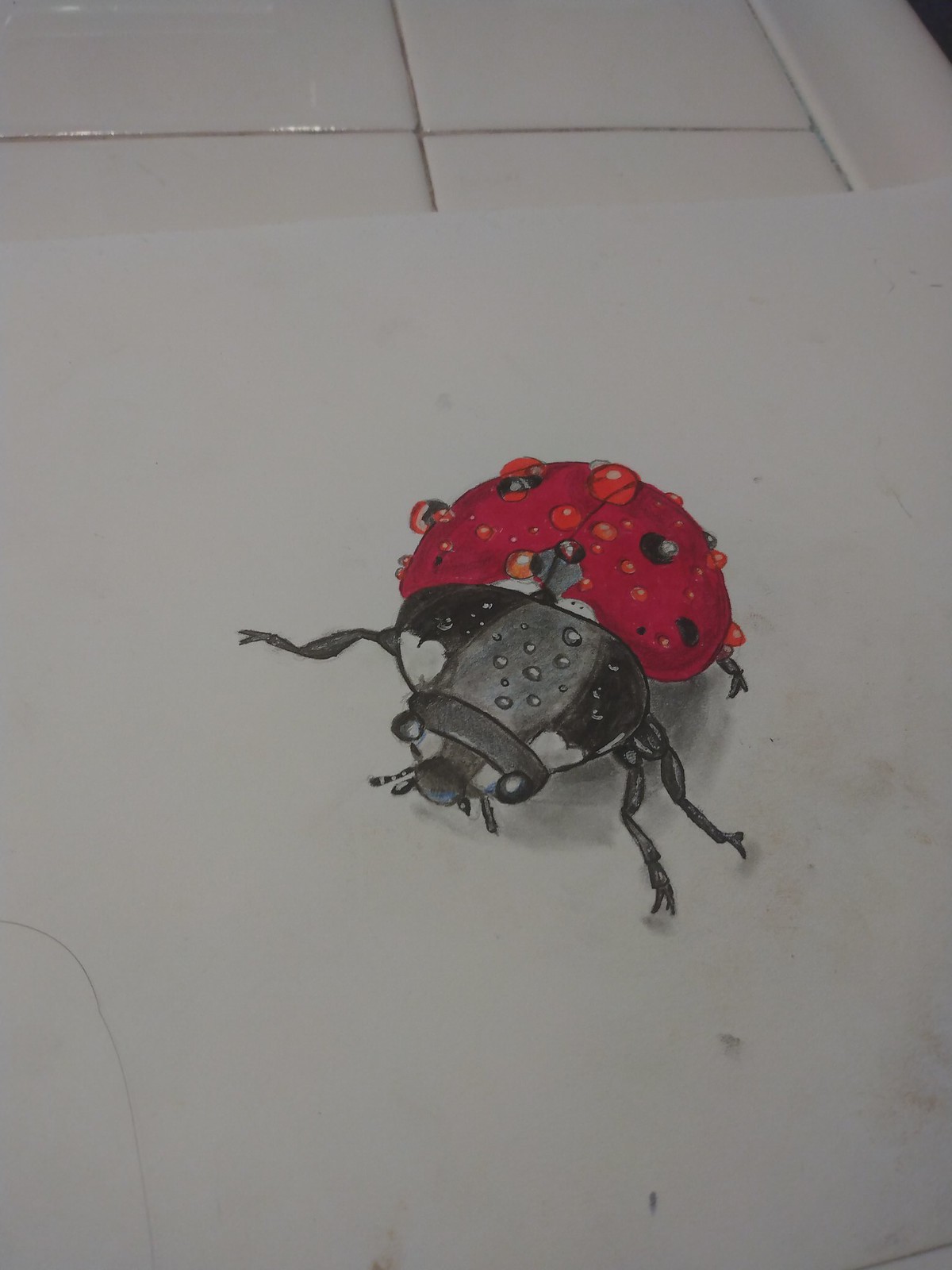In this image, we see a light gray, tiled floor serving as the backdrop. Laid across the floor is a light gray mat or towel. At the center of the composition is an insect that superficially resembles a ladybug. However, upon closer inspection, its appearance deviates slightly from the typical ladybug. The insect features an oval-shaped head with a small black nose and delicate antennae protruding from its front. There are four visible legs, all black, emerging from underneath its body. Its head is predominantly black with a hint of gray underneath. The insect's back, while flat and black, prominently showcases a vibrant red shell adorned with characteristic black spots. The shell is wet, with noticeable raindrops or water droplets clinging to its surface, adding texture and a touch of realism to the scene.